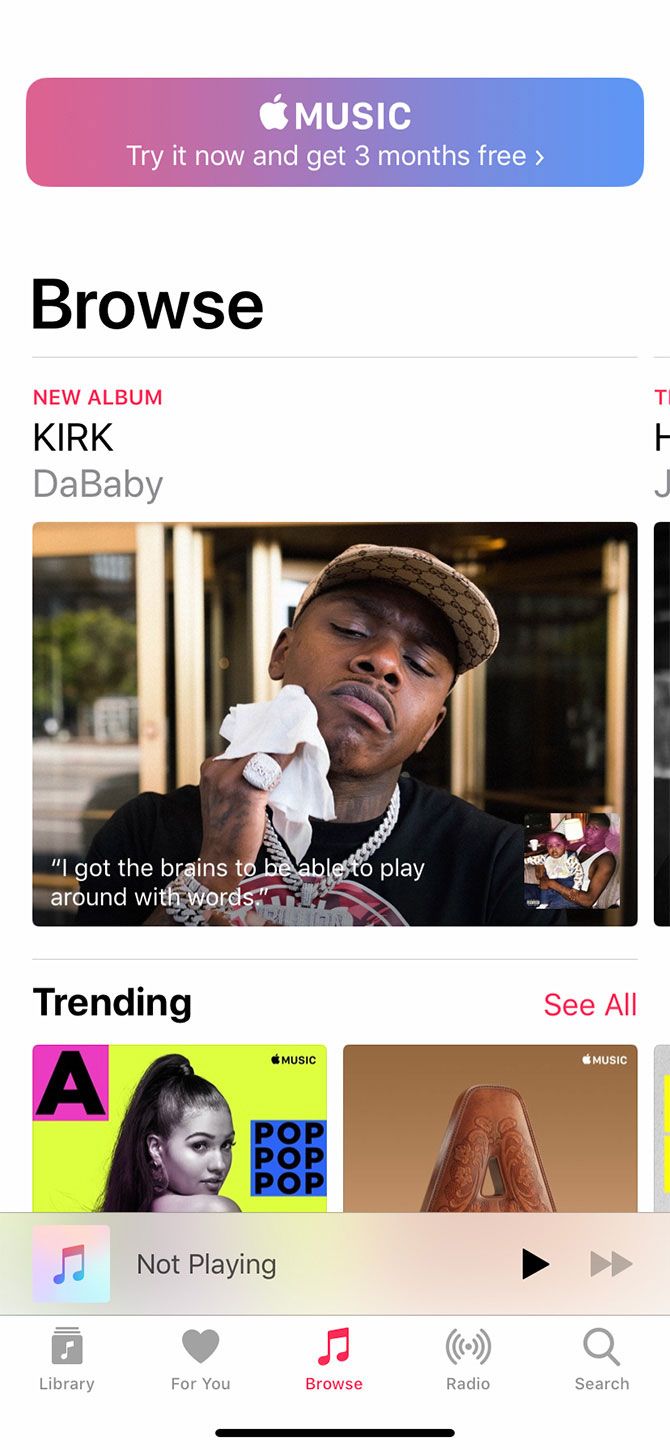The image is a screenshot of the Browse section in the Apple Music app. At the top of the screen, the Apple logo is prominently displayed next to the word "Music," followed by an invitation to "Try it now and get 3 months free." Below this header, on the left side, is the "Browse" tab. Directly beneath the "Browse" tab, there is a featured section highlighting a new album titled "Kirk" by DaBaby. The album feature includes an image of DaBaby and a quote from one of his songs: "I got the brains to be able to play around with words."

Adjacent to the album feature, on the right, is a "Trending" section where the word "Seahole" is displayed in a pinkish-red color. Below the trending section, the screen shows two cover photos, likely representing different playlists.

At the bottom of the screen, there is a control bar with "Not Playing" displayed, along with a play button on the right side and a fast forward button to its extreme right.